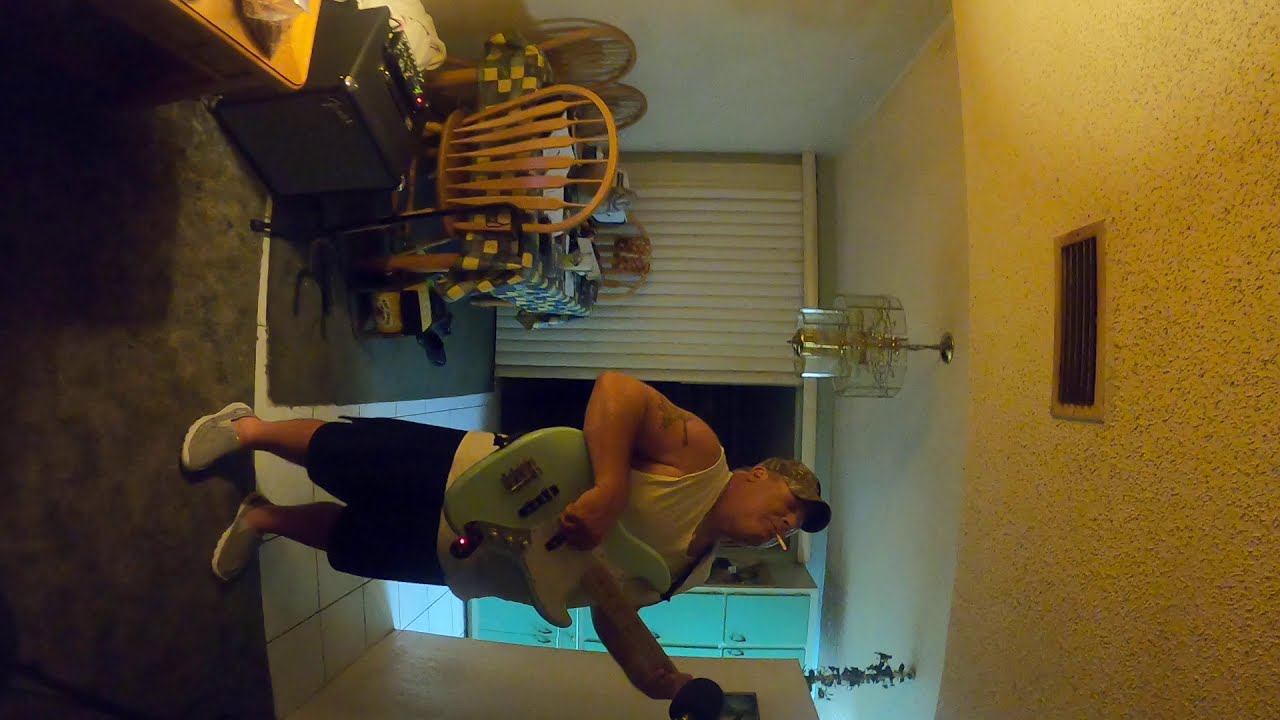The photo captures the interior of an apartment, slightly rotated so that the bottom appears on the left side. The focal point is a man standing and playing a mint-colored electric guitar with white accents. He is wearing a white tank top, black shorts, gray tennis shoes, and a gray hat. A cigarette dangles from his mouth as he focuses on his music. The man stands on a dark gray carpet, with a dark gray or charcoal amplifier next to him. In the background, dining furniture—including light-colored wooden chairs—is visible, along with a ceiling lamp and a balcony. The overall atmosphere is casual and homey, with the kitchen table adding a touch of lived-in warmth to the scene.